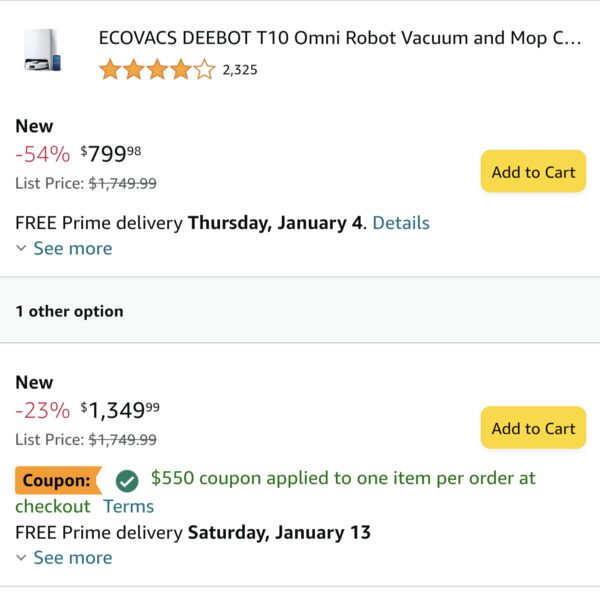The image depicts a section of an Amazon product listing for the Ecovacs Deebot T10 Omni Robot Vacuum and Mop Combo. The product boasts a four-star rating based on 2,325 customer reviews. It is currently being offered at a significant discount of 54%, bringing the price down from $1,749.00 to $799.98. Free Prime delivery is available, with an estimated delivery date of Thursday, January 4th. An "Add to Cart" button is prominently displayed.

Another buying option is also presented: a new unit at 23% off, priced at $1,349.00, with free Prime delivery estimated by Saturday, January 13th. Additionally, there is a green checkmark indicating a $550.00 coupon that can be applied to one item per order at checkout. This coupon makes the two prices nearly identical, with only a one cent difference after applying the coupon. 

Thus, the effective price for the Ecovacs Deebot T10 Omni appears to be around $800.00 after discounts and coupons.